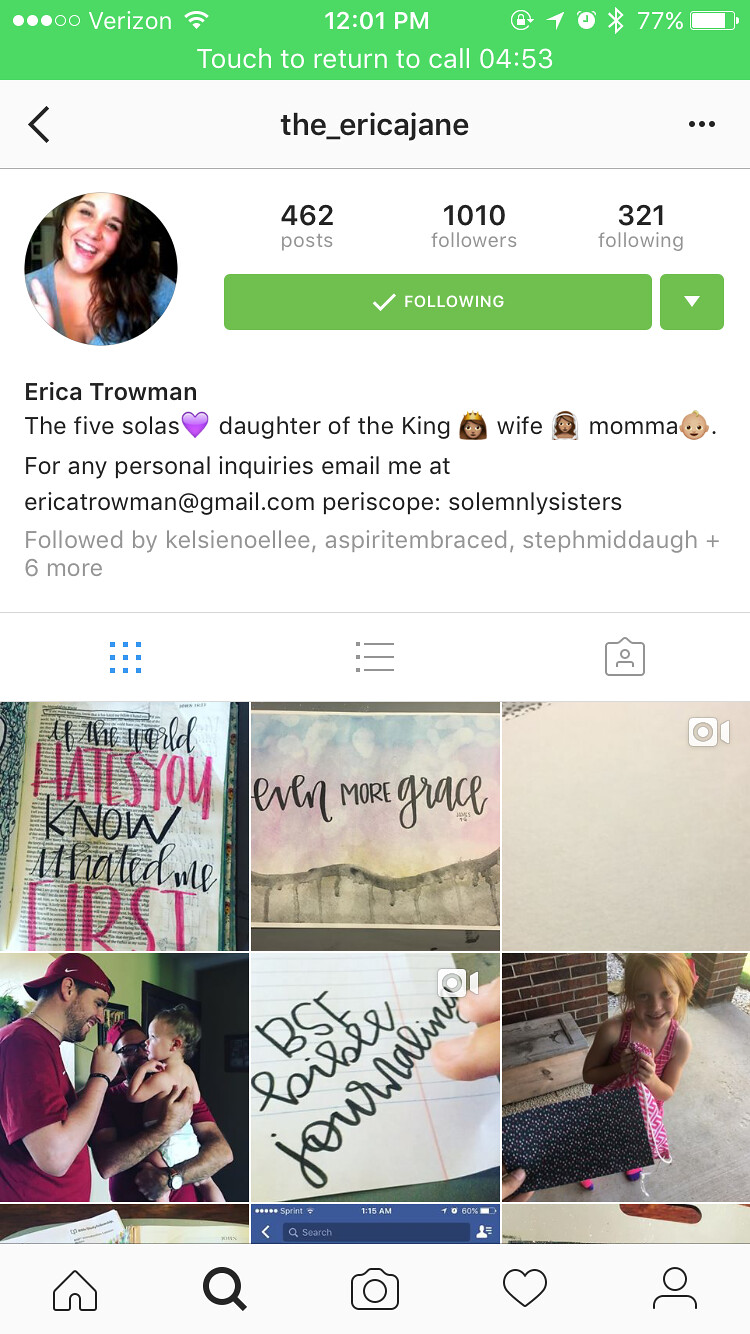This image is a detailed screenshot from a mobile device of an Instagram profile. At the top, the status bar shows the carrier as Verizon, the time is 12:01 PM, and the battery level is at 77%. A green bar indicates a call in progress, lasting 4 minutes and 53 seconds. The Instagram profile belongs to a user named TheEricaJane. The profile picture, located at the top left, features a girl. 

TheEricaJane, whose real name is Erica Troman, has made 462 posts, has 1,010 followers, and is following 321 others. The bio underneath her photo reads: "The five solas, daughter of the king, wife, mama. For any personal inquiries, email me at ericatroman@gmail.com," followed by references to "Periscope, solemnly sisters." The profile grid below the bio showcases a mix of quote images and personal photos, presumably of her family, including her daughter and husband. This is a modern, personal Instagram profile view, indicative of today's social media landscape.